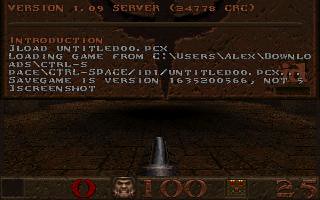Screenshot of a vintage game interface, version 1.09. At the top, it displays the word "Server" followed by the number "34778" in parentheses, along with "CRC" in parentheses. Below this, the term "Introduction" appears in light brown text, accompanied by white text underneath. The visual centerpiece features a sword emerging from the lower center of the screen. Additionally, a horizontal bar spans the bottom of the image from left to right.